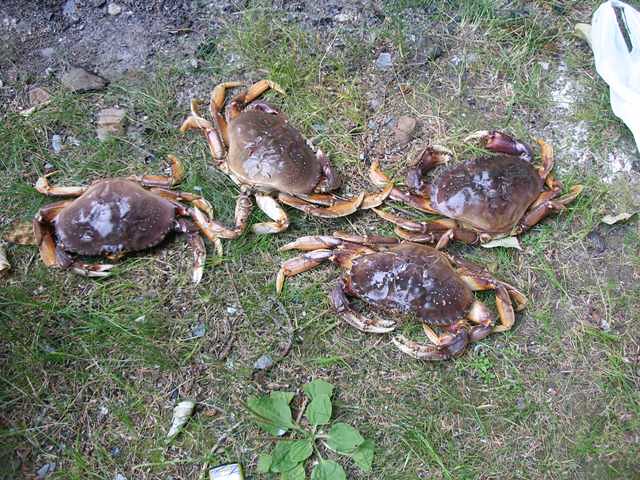A photograph taken from an overhead perspective captures a patch of very short, trampled grass interspersed with dirt and debris. Prominent in the scene are four crabs, placed on the ground in a specific arrangement. Three crabs lie horizontally across the top, while the fourth is positioned below them towards the right. The crabs feature dark brown or grayish-green shells with legs that exhibit a mix of tan, burnt rust, and white coloration, particularly noticeable near the claw areas. Some crabs face the camera, while others are oriented away or to the side. The ground below the crabs is littered with leaf debris and small twigs, with a notable weed located directly at the bottom center of the image. In the top corners, gray stones and a mysterious white object add texture to the background. Sunlight casts a reflection from the left, highlighting the crabs' shells.